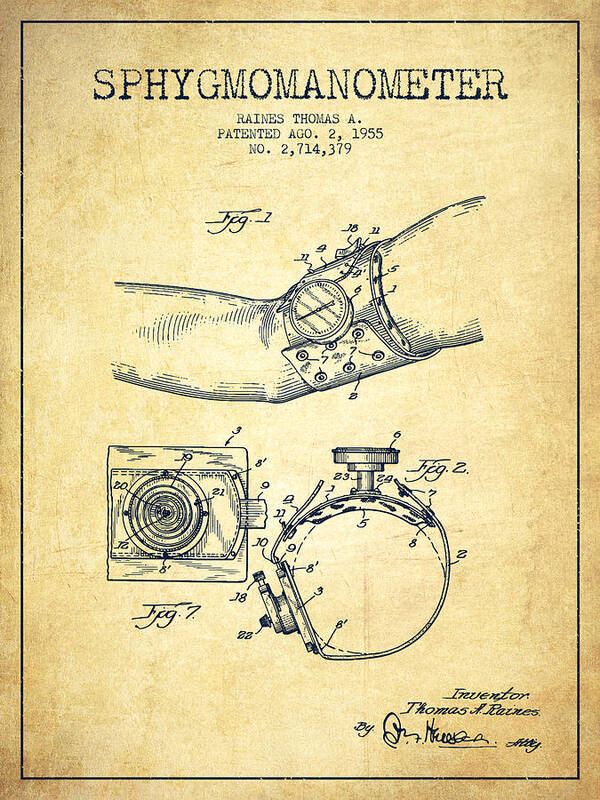This vertically aligned rectangular image resembles a page from an aged book with a beige-brown stained background, bordered in black. It prominently displays the word "SPHYGMOMANOMETER" at the top, followed by smaller text: "Reins Thomas A. Patented A.G.O. 2, 1955. Number 2,714,379." Hand-drawn figures illustrate the device: in one drawing, a person’s arm is shown wearing the instrument, which looks like a traditional blood pressure monitor with a cuff and a dial. A close-up of the dial is depicted below. Additional views, including a profile and what appears to be the back of the arm band, are also displayed. The inventor’s name, "Thomas A. Reins," along with his signature, is located at the lower right corner. The paper is aged, with brown and white hues, and the lines and font appear in a blue-black color.